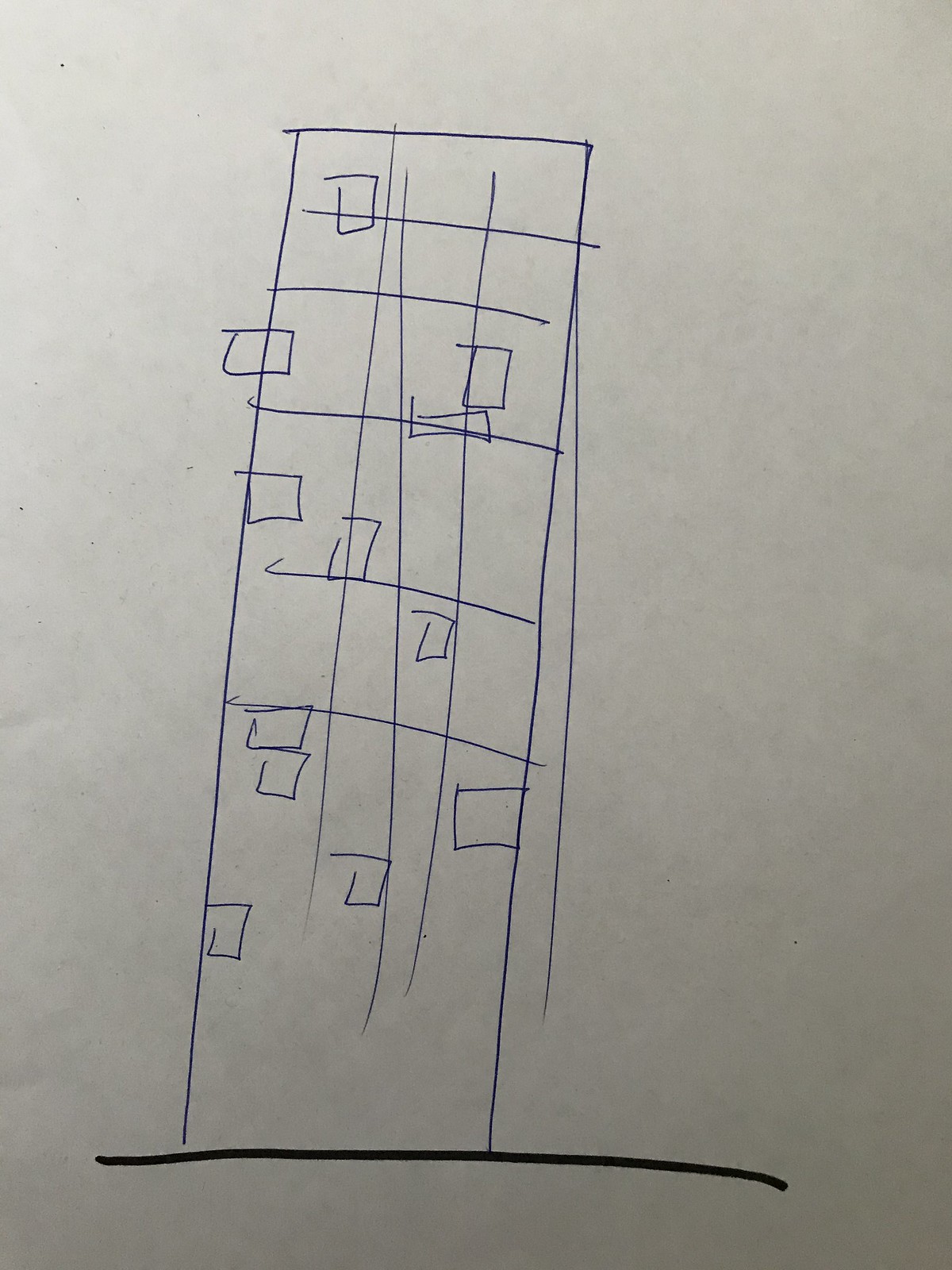The image showcases an up-close view of a rough drawing of a building, sketched with what appears to be a blue pen on a white piece of paper. The depicted structure is a tall, multi-story building, potentially with six or seven levels. The drawing features horizontal lines, five of which denote various stories of the building. Scattered throughout the building are 12 windows, some even intersecting with the horizontal lines, while others reside entirely within the designated stories.

In addition to the windows, three vertical lines are drawn, segmenting the building into three sections. Notably, one of these vertical lines is crooked. Another line runs externally along the building's left edge, stretching from top to bottom. The base of the building is reinforced by a solid black line, likely drawn with a marker, that runs horizontally across the bottom of the paper.